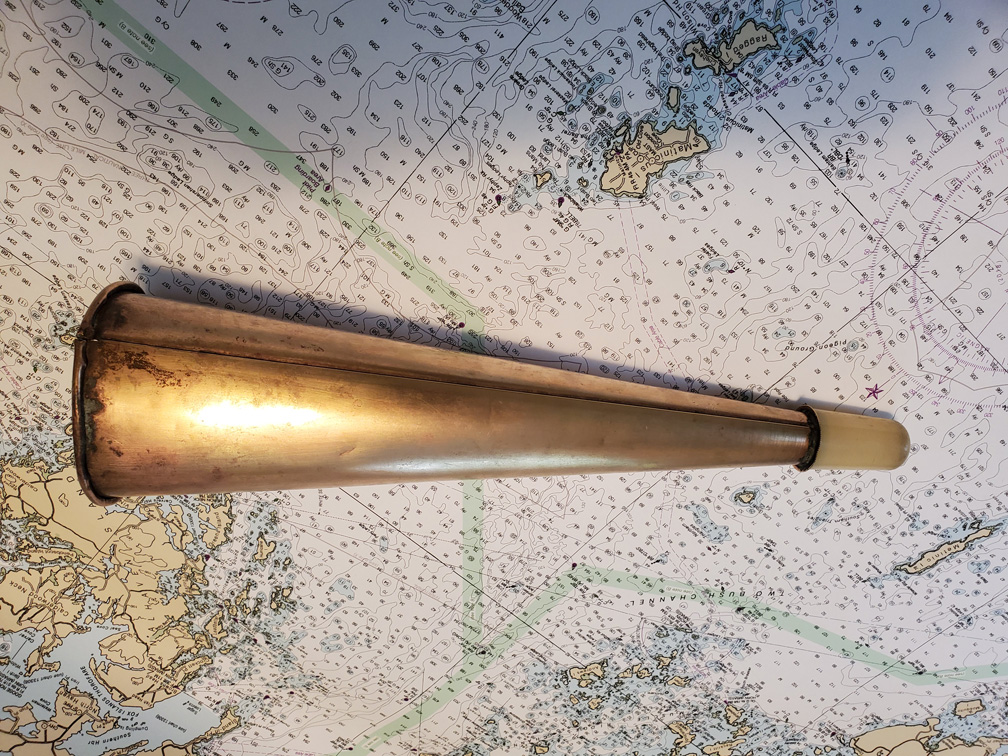The image features a vintage, brass-colored horn, resembling a bugle, with a narrow, white plastic-covered section at one end that broadens out into a thicker, circular form. This horn is affixed to a large map depicting various landmasses and islands. The map showcases several distinctive elements: at the top right, there's a cluster of islands; at the bottom left, a larger landmass is visible, and towards the center, we see a map logo. Scattered across the map are numerous numbers and outlined regions, which likely indicate ocean paths or shipping routes. The overall setting suggests that the brass instrument might have been used for navigation or communication on an old ship.